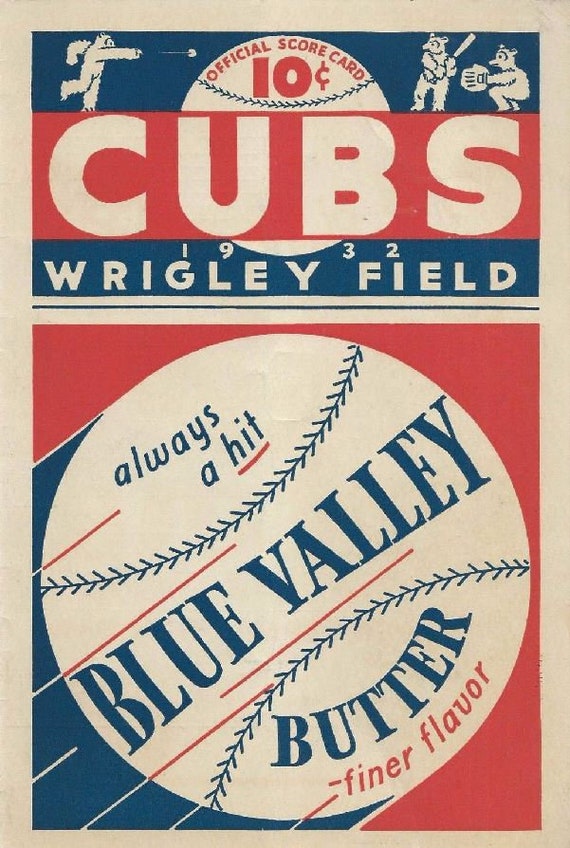The image is a photograph of a vintage baseball scorecard cover from 1932 featuring the Chicago Cubs at Wrigley Field. The poster has a light gray (or cream-colored) border framing a colorful and intricate design. At the top center, in bold red letters, it reads "Official Scorecard" followed by a large number "10" with a cent sign beside it against a dark blue background. 

On the left side, there is a white-colored bear pitching a baseball, while the right side shows another bear ready to bat with a stick and a third bear crouched behind as a catcher, decked out in a baseball glove, both depicted in a cartoonish, playful style.

Below this scene, a red rectangular box spans the width of the poster with the word "Cubs" in large white letters. Directly underneath, against a blue background, it states "1932 Wrigley Field."

The lower two-thirds of the poster prominently features a large white baseball detailed with blue stitching, and across its center in blue letters, it reads "Blue Valley." Below this, in red letters, is the phrase "Butter," and further beneath, also in red, is the tagline "Finer Flavor," suggesting an advertisement for Blue Valley Butter. 

This detailed depiction captures the essence of a classic piece of baseball memorabilia, reflecting both the sport's heritage and advertising art from the early 20th century.